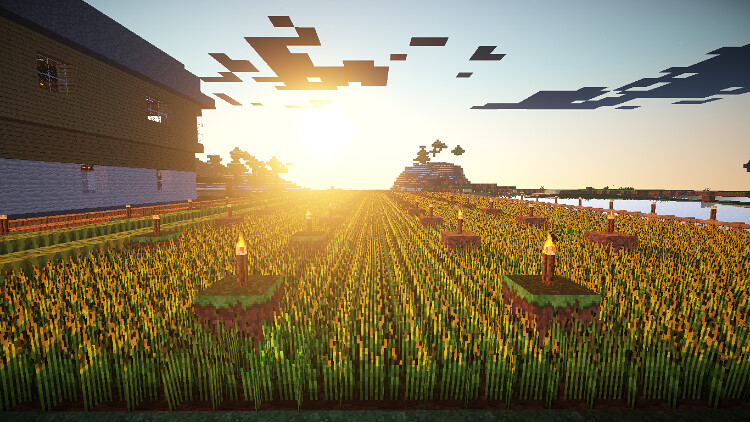The image depicts a digitally generated scene reminiscent of a computer video game. In the foreground, there is a vibrant field of flowers primarily in shades of green, interspersed with yellow sunflowers that have striking black centers. Scattered across the field are dirt mounds or podiums, varying in appearance—some adorned with a strip of green grass, others capped with just brown dirt. Certain podiums have flames emerging from brown cylindrical structures on top.

The sky above is a clear blue, but it is dotted with black, block-like structures that seem to float or hover. In the background, abstract trees add an artistic, surreal touch to the landscape. A body of water lies to one side of the image, adding to the scenic variety. On the opposite side, there is a brown and white building with a dark gray roof, partially obscured by surrounding shrubbery. The entire scene blends natural and fantastical elements, creating a uniquely immersive visual experience.